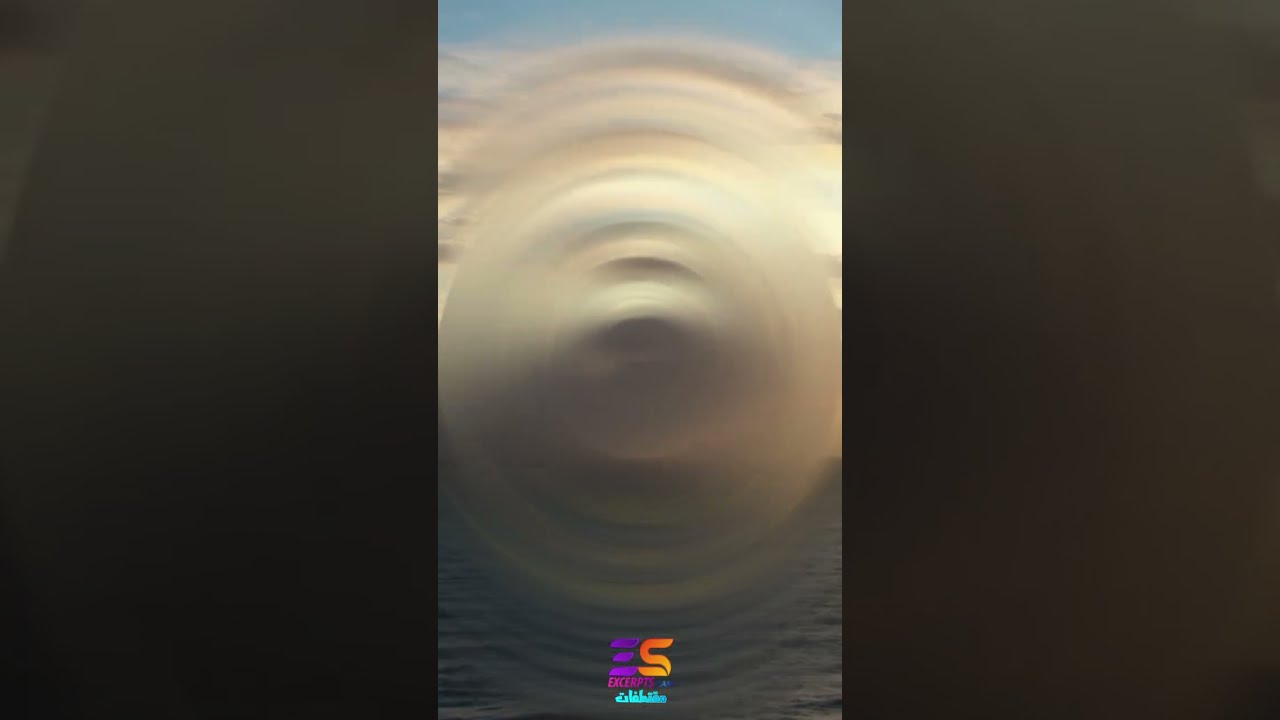The image is composed of a central vertical rectangular strip set against a larger horizontal black background. The central strip depicts a serene scene of the sea and sky, with the sea being dark blue at the bottom and the sky a light blue above, filled with scattered clouds. A spiral filter overlays the image, distorting it into a vortex shape that gives the illusion of swirling sand in a tannish-brown hue, possibly indicating a fast-spinning vortex. Midway through the image, the spiral effect merges both the sea below and the sky above, creating a dynamic and somewhat chaotic effect. At the bottom center of this central strip, a distinctive logo is positioned. It resembles the letters "E" and "S" with three vertical lines in blue to the left and an "S" in shades of orange and yellow. Beneath the logo, the text "excerpts" is clearly visible, suggesting this may be promotional or indicative of a brand. The very fine, unreadable text below "excerpts" adds a final touch to the detailed and layered composition.